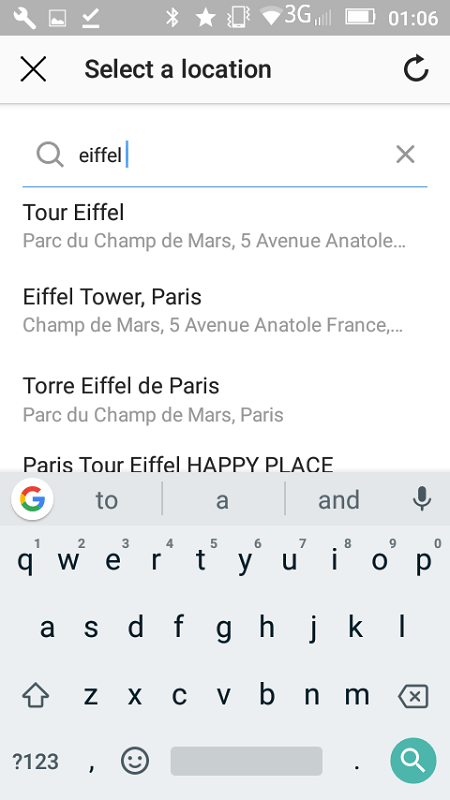The screenshot displays a typical cellphone interface with the following details:

1. A light gray status bar at the top displays the time (1:06), 3G connectivity, and a nearly full battery indicated by white icons.
2. Below the status bar, there's a light gray box that contains black font text reading "Select a location."
3. Directly beneath this box is a white search field, featuring a light gray magnifying glass icon on the left, and the text "Eiffel" (E-I-F-F-E-L) in black. A blue cursor follows the text, and there's an 'X' icon on the far right of the search field.
4. Moving down, a thin blue line separates the search field from the search results:
   - The first result is "Tour Eiffel" in bold, followed by "Parc du Champ de Mars" in lighter gray font, which is the address.
   - The second result reads "Eiffel Tower Paris," with another light gray address underneath.
   - Below, it says "Tour Eiffel de Paris" in black font, paired with its address below.
   - The final search result in bold states "Paris Tour Eiffel happy place."
5. At the bottom of the screenshot, there's a display of a Google keyboard featuring the Google 'G' symbol in the upper left corner. It is a standard cellphone keyboard layout.

This detailed screenshot captures the process of searching for the Eiffel Tower on a mobile device, showcasing various results and the typical layout of a smartphone interface.